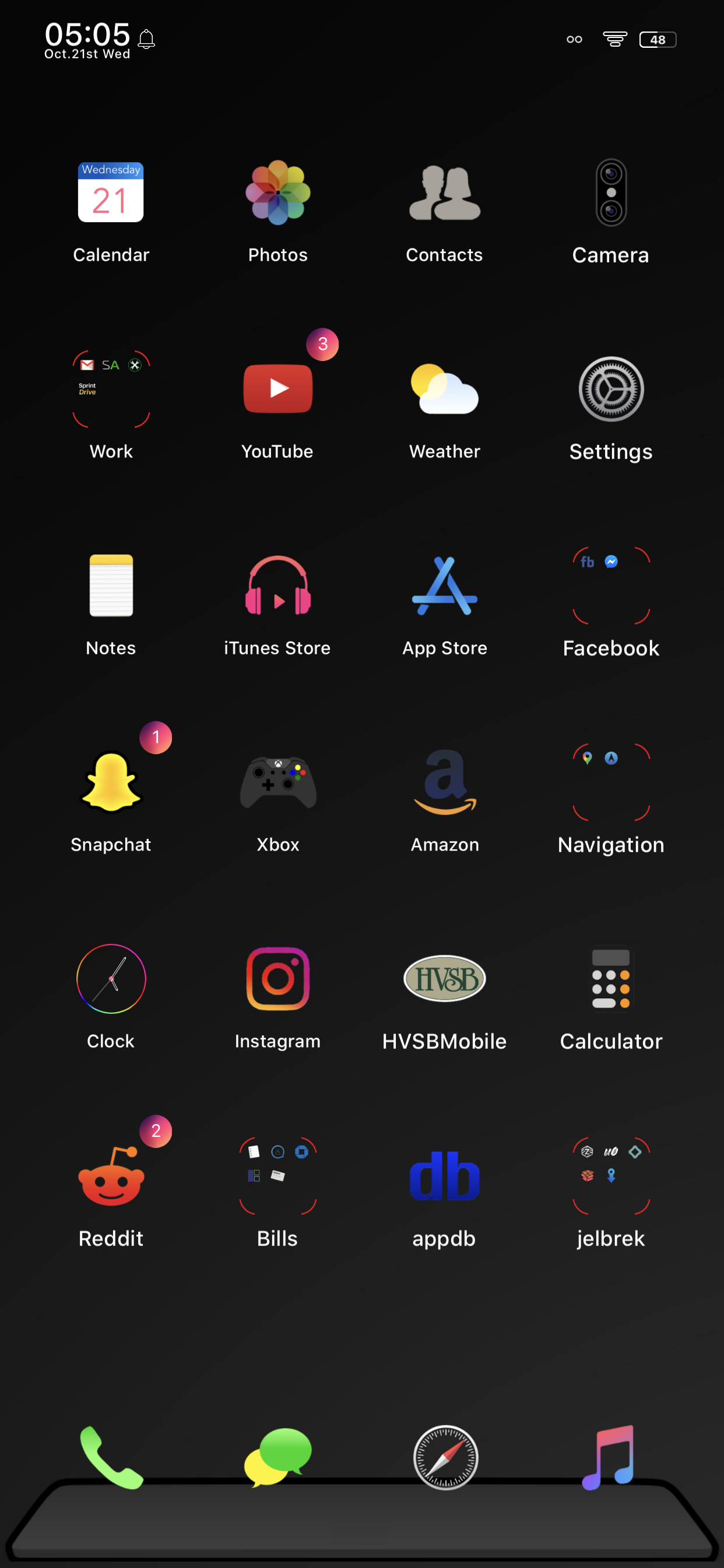The home screen of an iPhone is displayed, likely customized with a unique skin that emulates an older Android interface. The status bar at the top shows the time as 5:05 on Wednesday, October 21st, with standard indicators for signal strength, Wi-Fi, and battery life. The home screen icons include various apps: Calendar, Photos, Contacts, YouTube (displaying three notification badges), Snapchat (one notification badge), Reddit (two notification badges), AppDB, Xbox, Amazon, and Instagram. The dock at the bottom of the screen houses the Phone, Messages, and Music apps. Despite the initial confusion due to the skin, the presence of the Safari, iTunes, and Apple App Store icons confirms that this is indeed an iPhone.